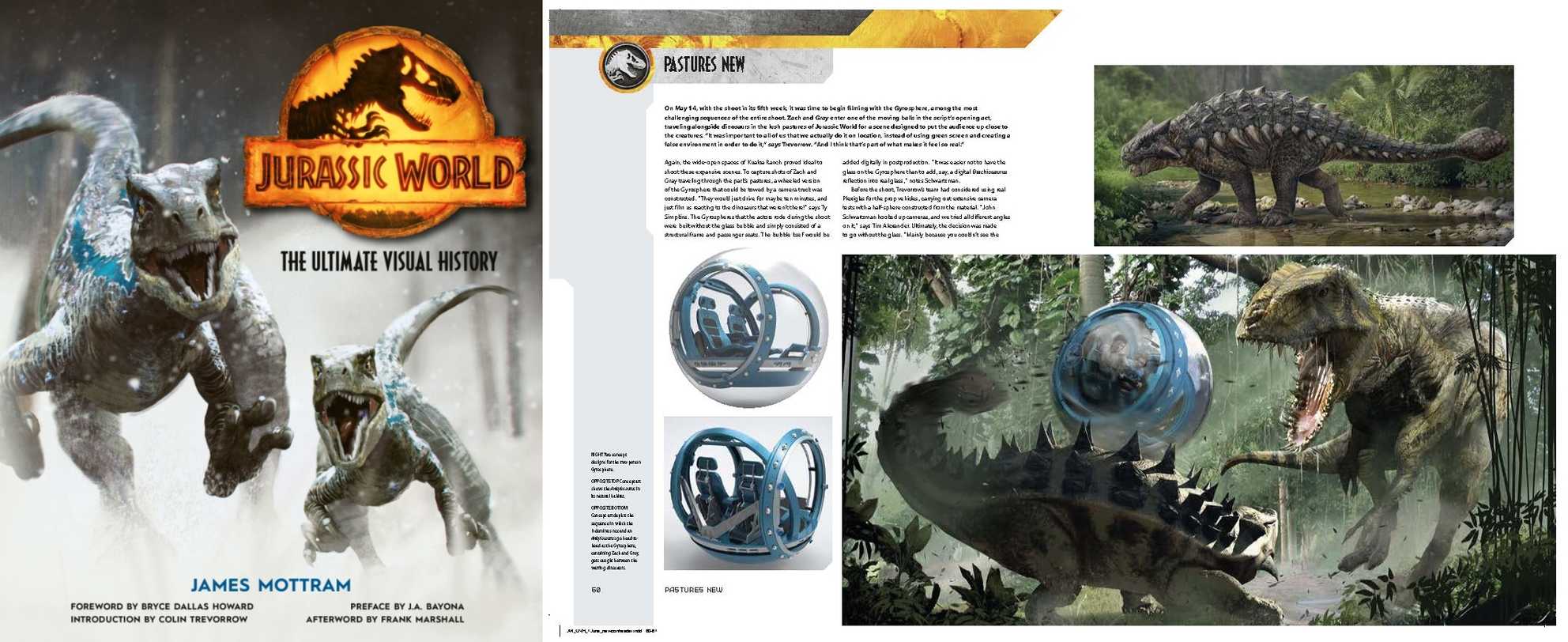The image showcases the cover of a book titled "Jurassic World: The Ultimate Visual History." Prominently featured is the Jurassic World logo, illustrating a profile of a Tyrannosaurus Rex skeleton with its mouth open. Below the logo, two grayish-blue Velociraptors with distinctive blue stripes along their backs are ambling towards the camera. These Velociraptors have sharp teeth and their mouths open, capturing a dynamic portrayal. The author, James Mottram, is credited in blue text beneath the Velociraptors, with additional black text that is too small to discern clearly.

To the right side of the image, there's a detailed mock-up of an interior two-page spread from the book. This spread includes paragraphs of text and concept art. One piece of artwork shows an ankylosaur among lush vegetation. Below this central illustration, another dynamic scene depicts an ankylosaur engaging in combat with a T-Rex, with a spherical observation unit – reminiscent of those featured in the Jurassic World movies – situated nearby. The observation unit, depicted in concept art to the left of the image, is a transparent, hamster-ball-like vehicle designed for viewing the park's dinosaurs up close. The scene is set within a dense jungle complete with vines and greenery, adding to the immersive atmosphere.